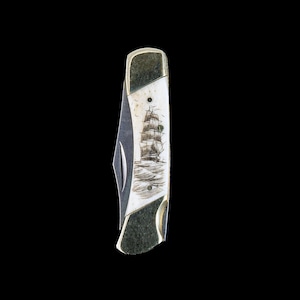The image features a square format with a dark black background. Centered within the square is a long, rectangular object that closely resembles a knife or razor. This object has a white central portion depicted with a detailed illustration of an early modern sailing ship on water. The top and bottom sections of the handle are characterized by a grainy black or dark gray shading, contrasting with the white middle part. Sticking out behind the central section is a grayish-white component, likely the blade, which appears curved and is situated on the left side of the object. Overall, the composition is monochromatic, with hues of black, white, and gray, and the entire image is text-free, focusing solely on the object in the center.